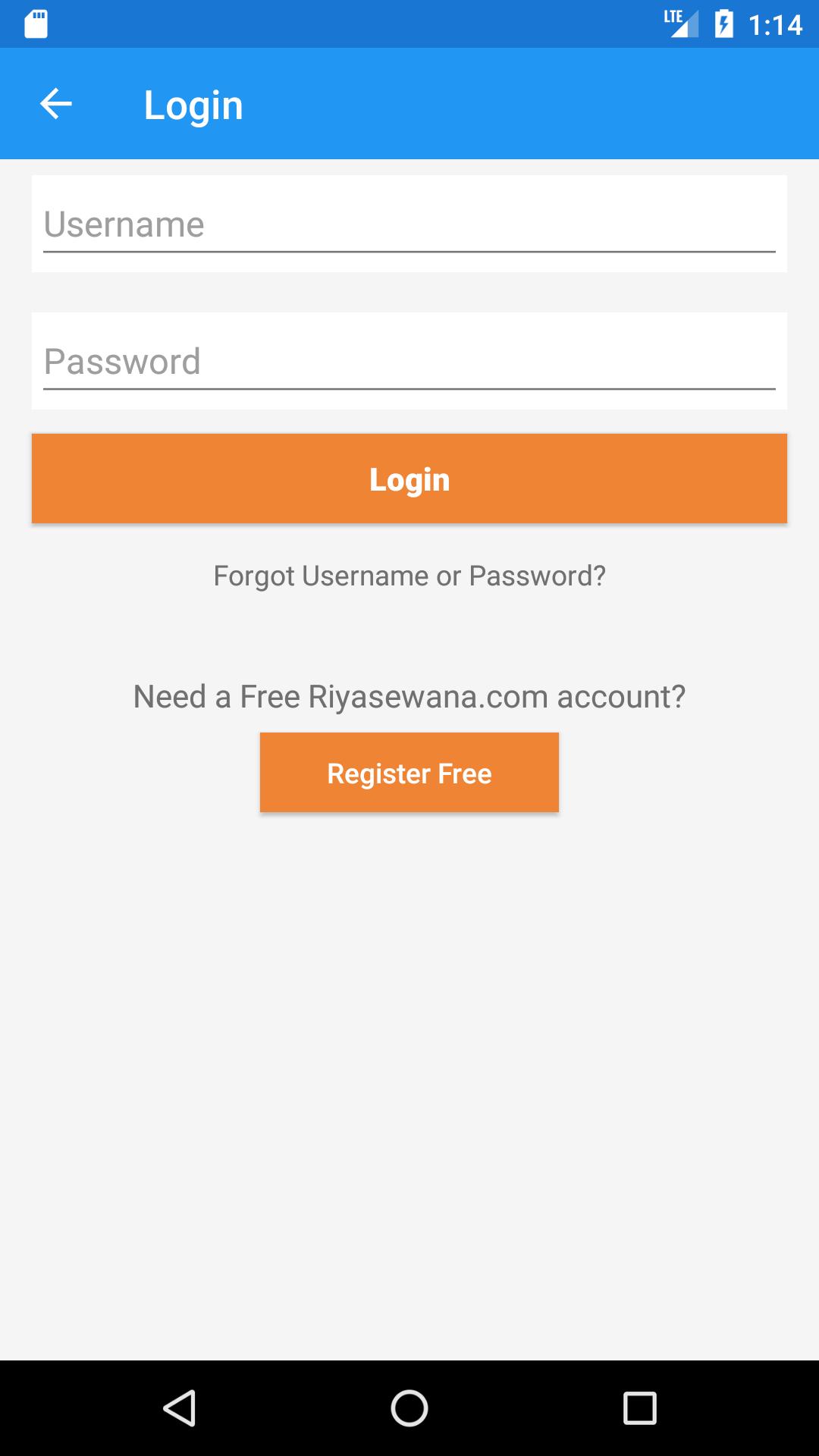The image is a screenshot from a smartphone displaying a login page for the riswada.com app. At the top of the screen, there is a blue status bar showing LTE connectivity, the battery percentage, and the current time. Directly below is a header with a white back arrow icon, and the word "Login" prominently displayed. 

The main body of the screen includes empty fields for "Username" and "Password," allowing users to input their credentials. Below these fields is an eye-catching orange "Log In" button. Additionally, there’s a "Forgot Username or Password?" link for users who need assistance with their login details.

Further down, the page invites users without an account to "Need a free riswada.com account?" followed by a "Register Free" button for new user registration.

The background of the page is predominantly white, providing a clean and simple interface, while the header with the title "Login" is set against a blue backdrop. At the bottom of the smartphone screen, there is a black navigation bar featuring three buttons: a back arrow on the left, a circular home button in the center, and a square-shaped multitasking button on the right, indicating typical smartphone navigation controls.

Overall, this image clearly represents the login interface of the riswada.com app, designed for mobile use.